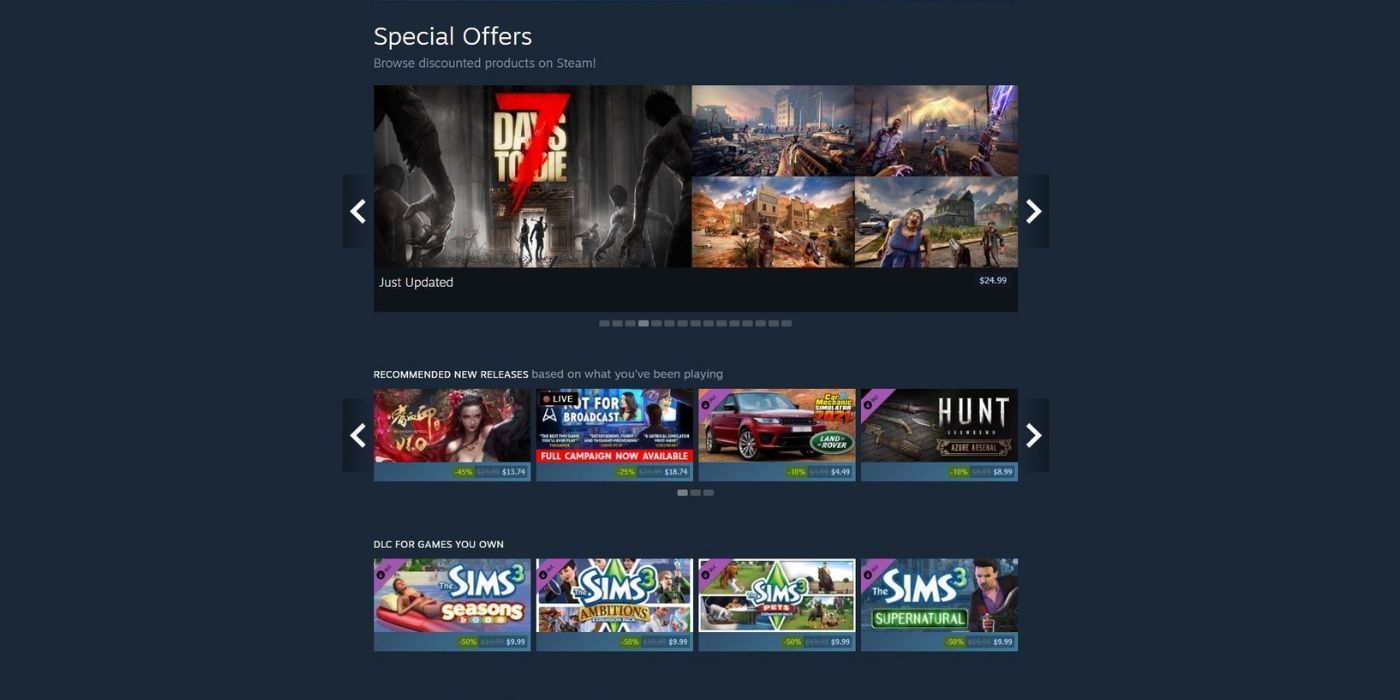The screenshot captures a store page within an application, set against a dark blue background. Dominating the top left corner, large white text announces "Special Offers," with smaller text below it exclaiming, "Browse Discounted Products on Steam!" 

Beneath this header, the page features a series of product showcases arranged in various formats. Prominently displayed is a large rectangular banner that stretches almost the entire width of the page. This banner features a navigational element: a white left-pointing arrow situated over a gradient background that transitions from very dark blue on the left to the background's dark blue on the right, and vice versa on the opposite side of the rectangle.

The main content of the rectangle showcases the game "7 Days to Die." On the left side, a double-height image depicts a grey forest with a bright doorway at its base, flanked by various grey zombies. Hovering above the image in distressed, yellowed font, the title reads "Days to Die," with a large "7" styled to resemble smeared blood overlaying the text.

To the right of this main image, a quadrant of four smaller screenshots presents various post-apocalyptic scenes featuring zombies and overcast skies, collectively matching the height of the left-hand image.

At the bottom of this large rectangle, a black strip spans its entirety. "Just Updated" is declared in white text on the top left of this strip, while the price "$24.99" is displayed in smaller white text on the top right.